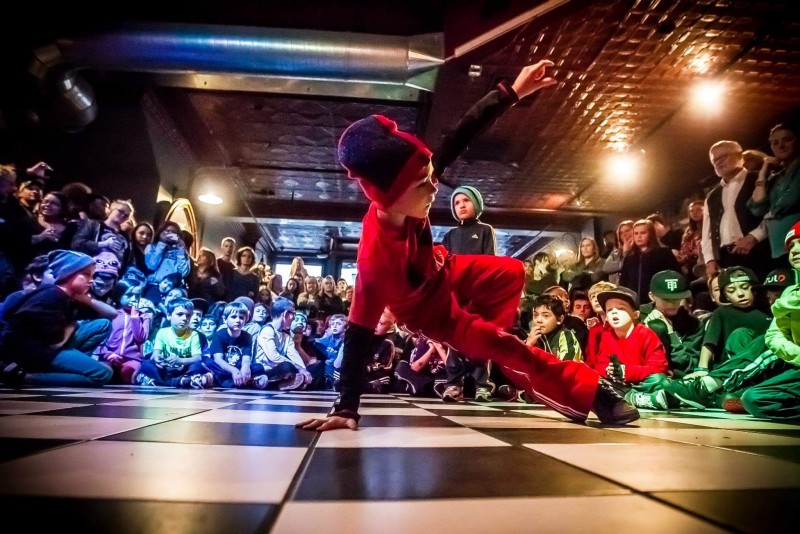Indoors, a dynamic photograph captures a young boy mid-breakdance on a black-and-white checkered tile floor. Dressed in a vibrant red outfit with black sleeves, black shoes, and a matching red and black wool cap, the boy is striking a dramatic pose. He balances on his left hand and foot, with his right leg and hand suspended in the air, showcasing his breakdancing skills.

Surrounded by a large, captivated audience of children and adults, the scene is both energetic and vivid. The children seated in a circle around the performer are bathed in contrasting blue and green hues due to overhead lighting, which creates a vivid and colorful atmosphere. Behind the seated children, additional kids and adults stand, all intently watching the young dancer. Among them, another child, dressed entirely in black, stands out, seemingly another dancer awaiting his turn.

The room's tin ceiling and warm, yellow lights cast a vibrant glow over the scene, enhancing the lively and communal vibe of this apparent hip-hop dance class or event. Every detail—from the checkered floor to the dance attire—adds to the rich tapestry of this dynamic and captivating moment.